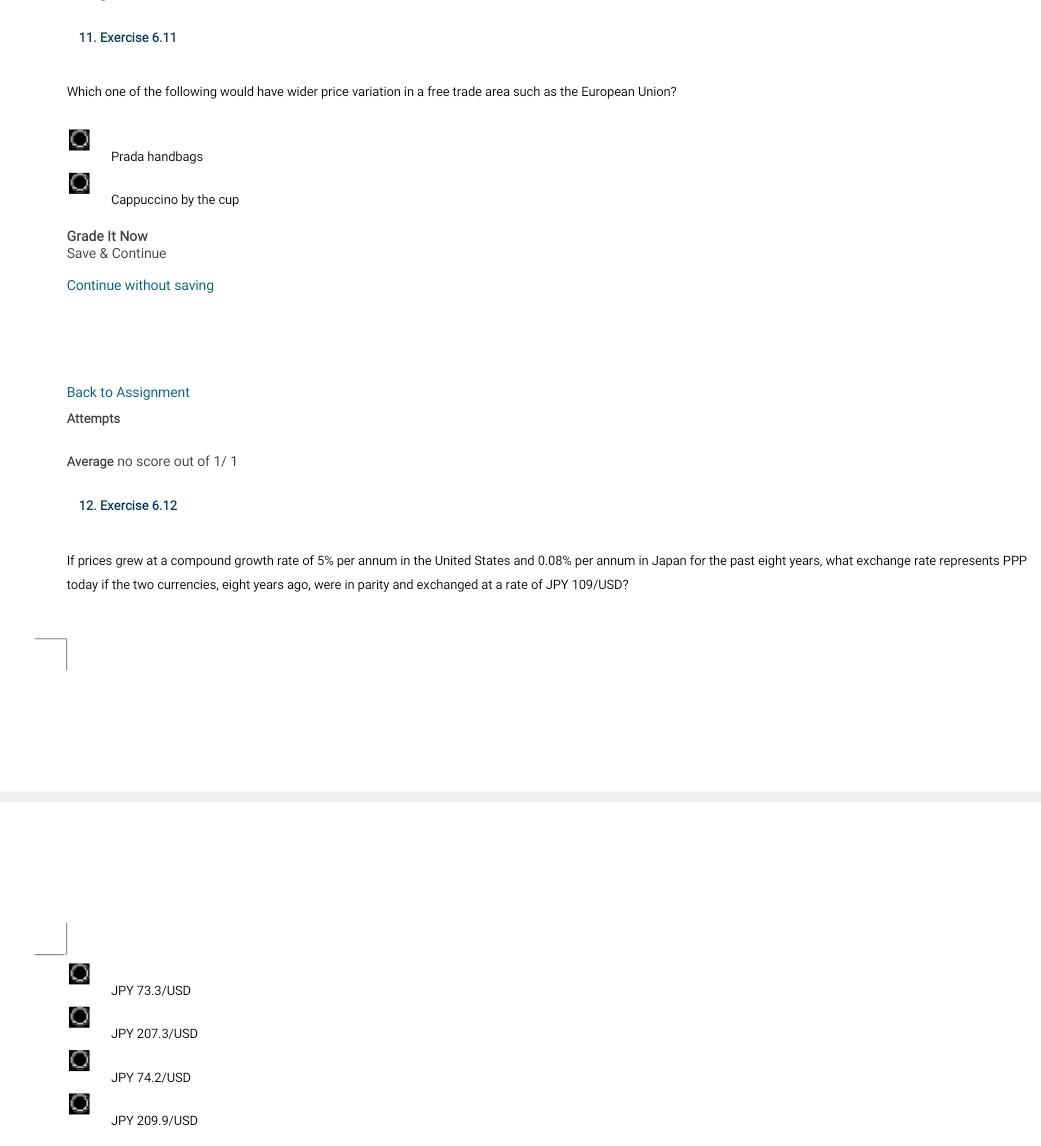This is a vertically oriented image captured from a computer screen, featuring a clean white background that creates a minimalist look typical of many online interfaces. The content displayed appears to be part of an online assignment or exercise, most likely from an educational platform.

In the top left corner, highlighted in blue, the text reads "11 Exercise 6.11." This is followed by black text posing a question: "Which of the following would have wider price variation in a free trade area such as the European Union?" Below this question are a few selectable options including "Prada handbags" and "Cappuccino by the cup." Additional options underneath include buttons labeled "Grade it now," "Save and continue," and "Continue without saving," the latter two highlighted in blue.

Further down, more text in blue indicates "Back to assignment," while next to it in black is the word "Attempts," along with information showing "Average, no score, 1 out of 1." Following this, in blue, is the label "12 Exercise 6.12."

A subsequent question in black reads: "If prices grew at a compound growth rate of 5% per annum in the United States and 0.08% per annum in Japan for the past eight years, what exchange rate represents PPP today if the two currencies eight years ago were in parity and exchanged at a rate of JPY 109/USD?" At the bottom of the page, various options are provided with differing JPY/USD exchange rates for selection.

The image clearly documents an interactive segment of an online module, showcasing questions focused on economic principles and currency exchange rates within different global contexts.